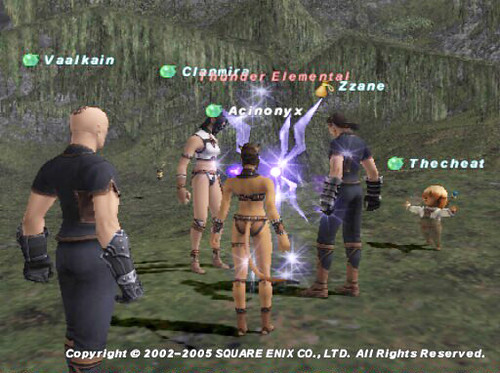The image appears to be a screenshot from a video game, evidenced by the visible copyright text at the bottom which reads "© 2002-2005 Square Enix Co., Ltd. All rights reserved." 

On the left side of the image, a distinctive male character with a bald head and light-colored skin is prominently featured. This character is donned in a tight black shirt that accentuates his muscular and strong arms, which are clad in black gloves extending up to the elbows. He also sports black pants. Above him, the name "Vaalkain" is rendered in bold text.

To the right of this character, two female characters are showcased, both wearing bikinis and possessing tails. One of them is also seen wearing short brown boots.

Dominating the center of the image is a dramatic purple light with emanating purple lightning bolts. The text "Thunder Elemental" is prominently displayed above this electrifying scene.

Adjacent to this is another character dressed in a black shirt and matching black pants, complemented by tall gloves. The name "Zzane" is written above this character.

Lastly, a diminutive character, a couple of inches tall with an orange head, is also present in the image. The text "The Cheat" is displayed next to this small figure, accompanying a green jewel situated to the left of it.